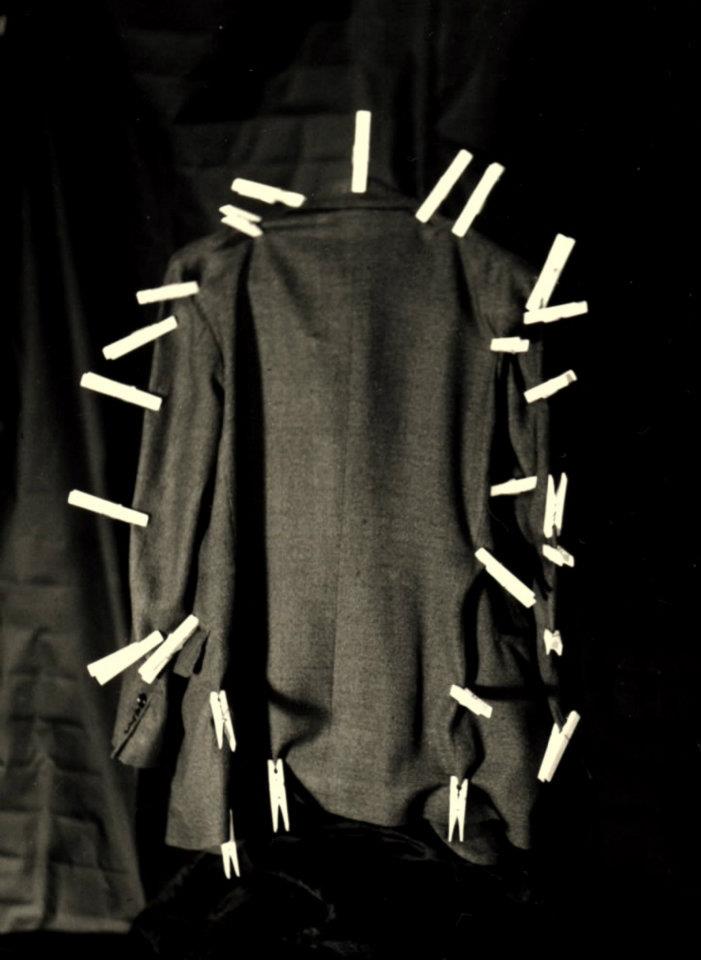This black and white photograph captures a dark grey or black men's dress coat, elegantly hanging with its back facing the camera. The scene is shrouded in darkness, with a single light source softly illuminating the coat's center. Intriguingly, the coat is adorned with an array of wooden clothes pins, lending an air of abstract art to the composition. The pins, numbering between twenty to thirty, are meticulously clipped around the entire perimeter of the coat, with no pins affixed to the back panel or bottom hem. Each sleeve is heavily decorated with about nine or ten pins, while the top and shoulders each bear one or two pins. The clothes pins, crafted from wood and metal, appear to serve no functional purpose and are positioned in a seemingly random arrangement, enhancing the artistic mystique of the image.